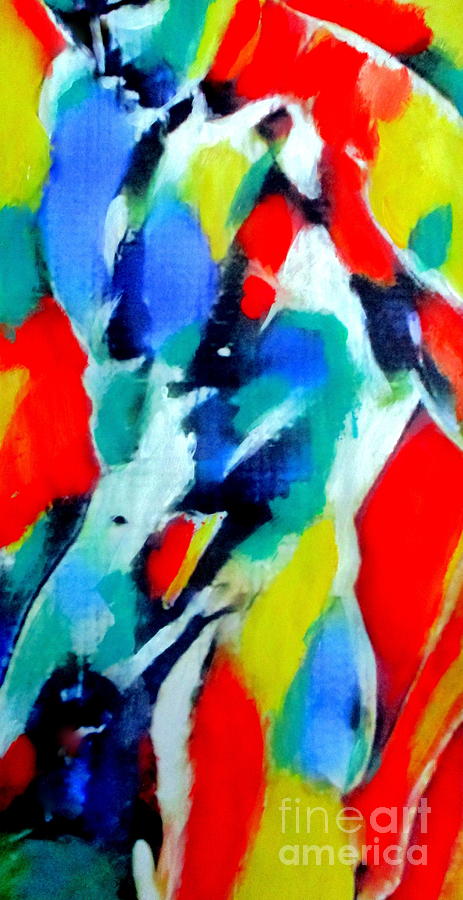The image is an abstract painting prominently featuring the naked physique of a muscular man. This modern art piece showcases a dynamic spectrum of colors including white, shades of gray, blue, yellow, dark blue, red, and even hints of greenish-blue and black. The man's body is painted with remarkable detail: his face appears to be looking down, his neck and left clavicle are painted red, his left deltoid is yellow, and his chest predominantly blue with traces of yellow. The background of the painting is dominantly red, interspersed with various splashes of blue and yellow. The composition includes streaks and splotches of color arranged in a woven pattern, with horizontal paint streaks running from top to bottom. In the bottom right corner, the signature "Fine Art America" is inscribed in light white letters, adding a touch of authenticity to this striking artwork.